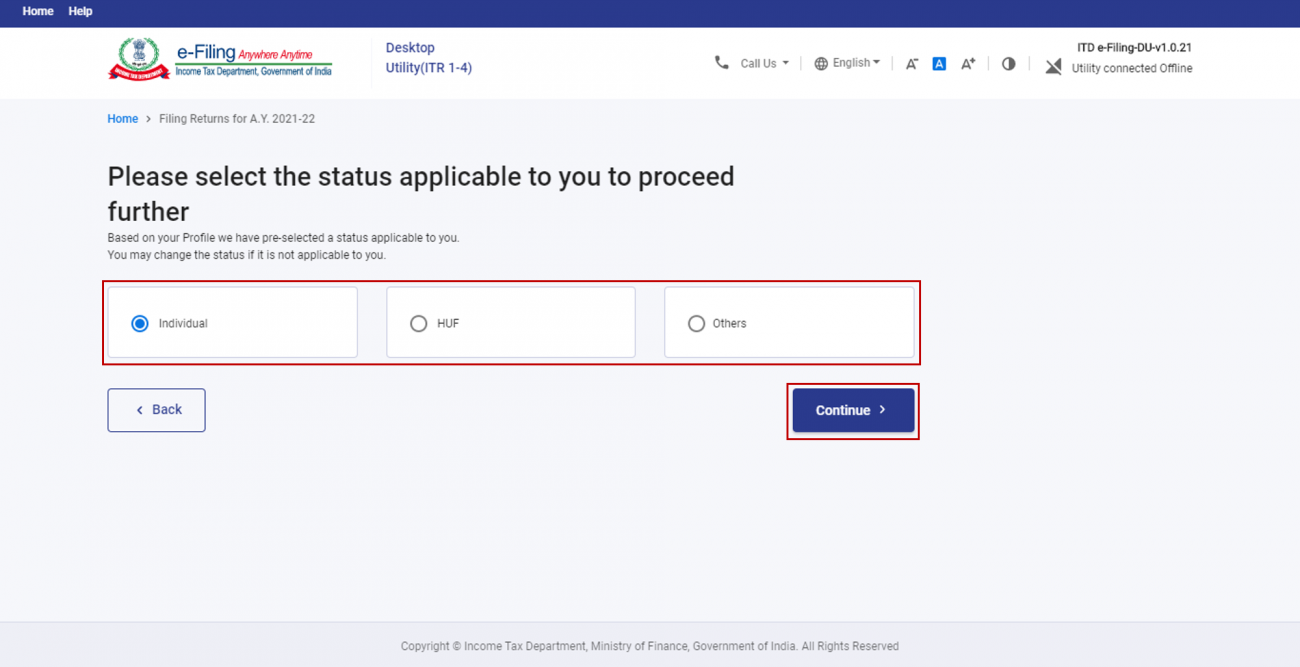The image is a cropped screenshot from a Government of India Income Tax Department web page. The top portion of the image features a narrow, dark blue navigation bar with two buttons labeled "Home" and "Help." Just below this bar, the web page's logo is prominently displayed, emphasizing its official nature. On the top right corner, there are various functional icons including a phone icon accompanied by "Call Us," indicating available customer support. The page is set to the English language, and there are options to adjust the font size and toggle between light and dark modes for better accessibility.

Dominating the main portion of the screenshot is a form with a grey background. This form features three radio buttons, each enveloped by a red border, signifying their interactive nature. The radio button options are labeled "Individual," "HUF," and "Others," with "Individual" being pre-selected. At the bottom of the form, there are "Back" and "Continue" buttons for navigation.